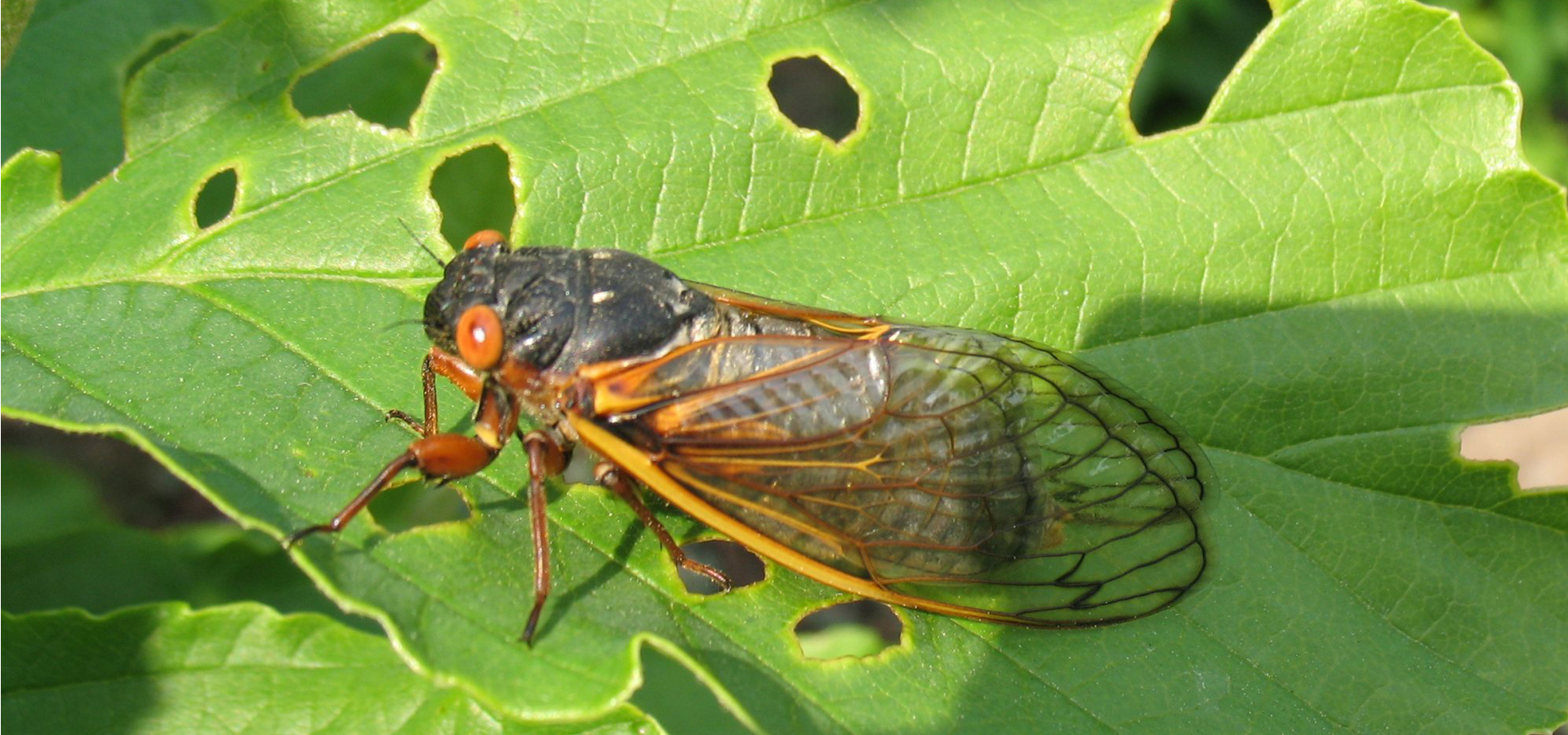This color photograph, taken in daylight, showcases a striking close-up of a black-bodied insect perched on a large, light green leaf. The insect's most prominent feature includes its large orange eyes, each adorned with a tiny white dot in the center. Its semi-transparent wings, extending toward the bottom right, reveal intricate dark brown veins and edges, with a faint yellow line near the bottom. The insect is gripping the leaf with its multiple brown legs, which include a few dark bends and black segments. The leaf itself displays a delicate network of fine and zigzagging veins, overlaid with larger veins running horizontally. Notably, the leaf has several holes, the largest of which is an oval shape located in the upper right quadrant. This rich detail captures both the beauty and complexity of the natural scene.